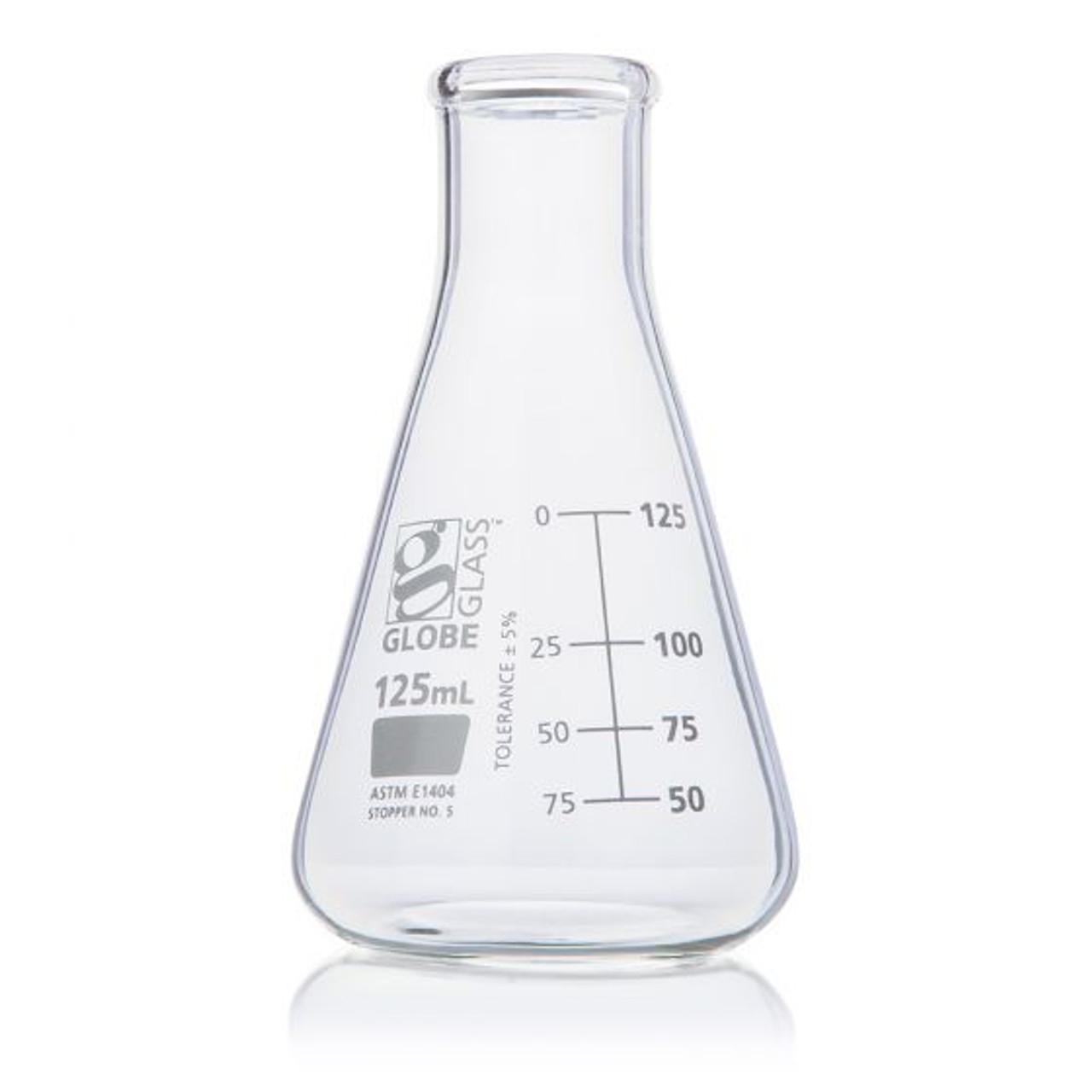The image depicts a scientific beaker commonly found in chemistry labs. The beaker has a wide base that tapers into a triangular shape as it reaches the top, ending with a lip reminiscent of an old glass milk bottle. It features notches and measurements on both sides: on the right side, the markings read 50, 75, 100, and 125 milliliters from bottom to top, while on the left side, the measurements are 0, 25, 50, and 75 milliliters from bottom to top. Additionally, the beaker is adorned with a logo that includes a large "G" and the words "Globe Glass." Beneath this logo, it prominently displays "125 ml," followed by a gray rectangle that reads "ASTM E-1404" and "Stopper No. 5." The beaker is notable for its rounded edges at the base and is typically used for mixing or holding chemical substances.